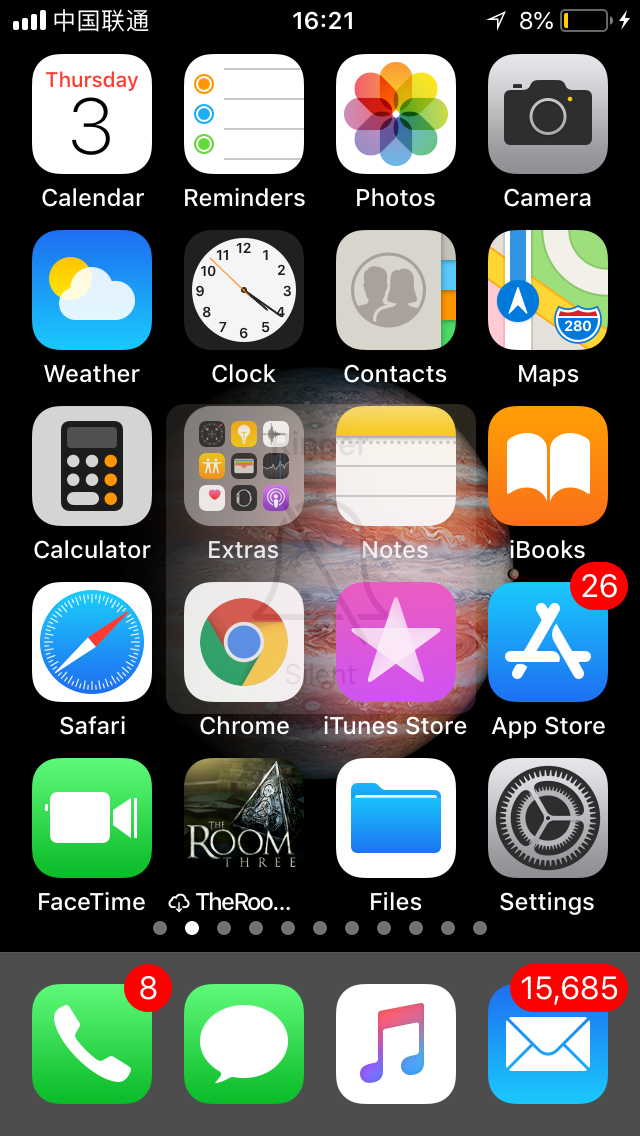The image is a screenshot from an iPhone with a predominantly black background. The central feature of the wallpaper is a captivating image of Jupiter, slightly below the center of the screen. 

At the top-left corner, there's a cellular signal strength icon with four white bars that progressively get larger. Adjacent to it are some Asian characters, possibly Chinese. The time, displayed in the middle at the top, reads "16:21". On the top-right corner, a white arrow pointing upwards to the right, which is hollow black in the middle, indicates that location services are active. Next, the battery indicator reads "8%" with the battery icon showing minimal charge filled in yellow, accompanied by a white lightning bolt indicating it's charging.

The screenshot shows various app icons prominently. The top-left app is the Calendar, marked by a white background and a big red "3" indicating the date is Thursday. Below the icon, “Calendar” is written. Due to the sheer number of icons, not all are listed, but the bottom row stands out with a grey background strip. From left to right, there's a green Phone icon with a white phone symbol, marked by a red dot with the number "8" indicating missed calls or notifications. Following the Phone icon, there's a Messages icon, a Music icon, and a Mail icon.